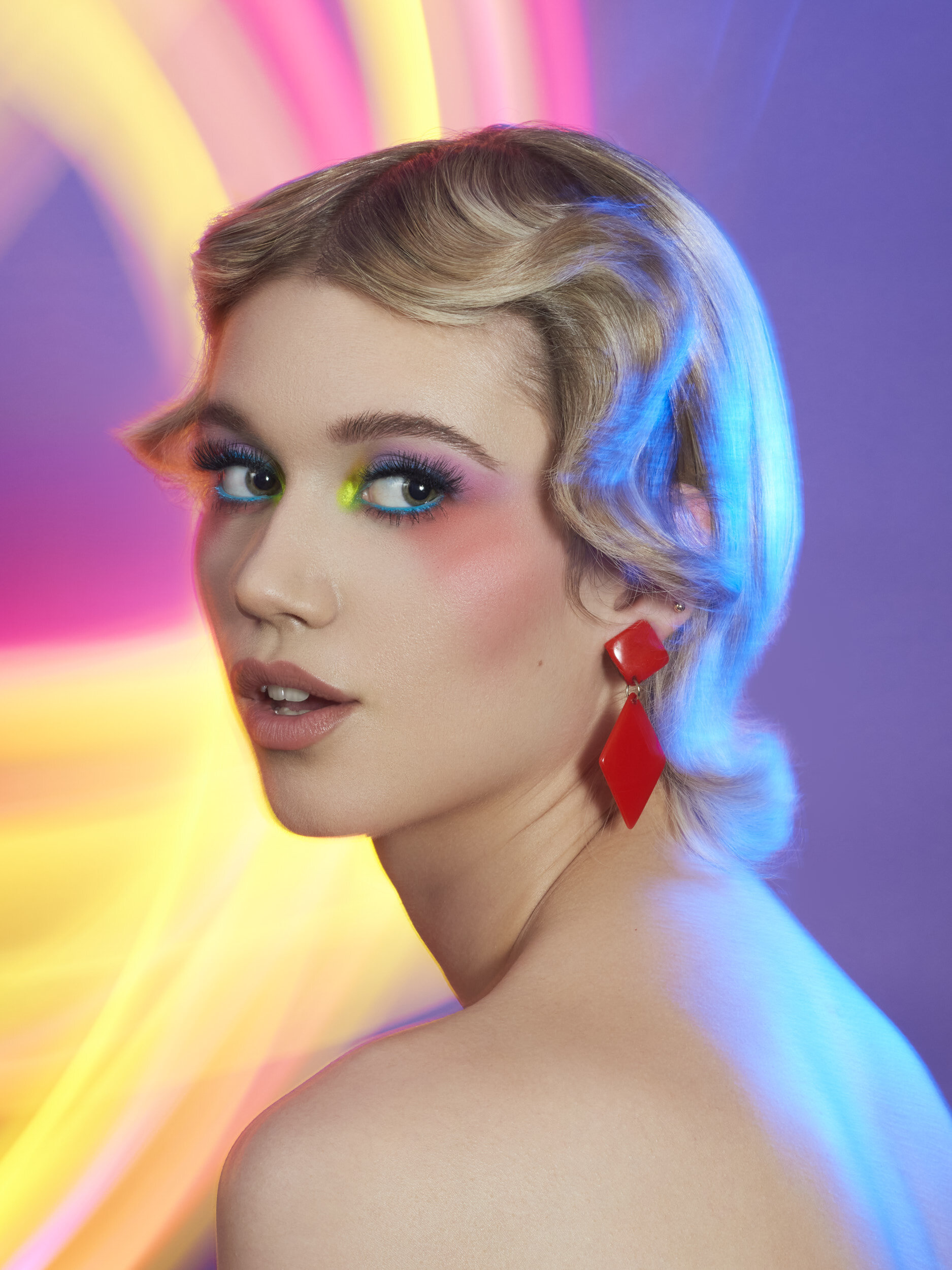The image portrays a young white woman, possibly in her mid-20s, with a radiant and cheerful expression as she looks directly at the camera. Her body faces away from the camera, but she turns her head over her left shoulder, engaging the viewer with her gaze. She dons a 1930s Hollywood glamour-inspired updo, featuring short, wavy blonde hair. Her makeup is vivid and dramatic, with neon eyeshadow in shades of blue, green, purple, yellow, and pink. Her cheeks have a rosy hue, and her lips, accentuated with lipstick, are slightly parted, revealing her teeth. She wears bright red, geometrically shaped dangle earrings, which could be described as a combination of square and triangular or two-prism-shaped. The background of the portrait is vibrant and psychedelic, showcasing swirling patterns of purple, pink, and yellow, which appear to be superimposed rather than part of the original setting. The overall impression of the image is soft and stylized, reminiscent of Taylor Swift's aesthetic.